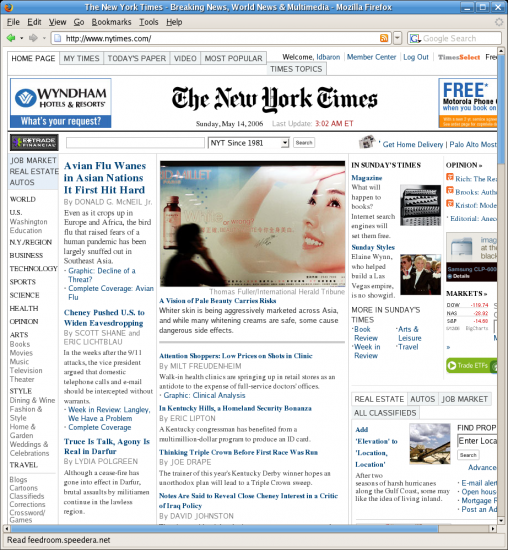Displayed on the screen is a Mozilla Firefox window open to The New York Times website. The tab is labeled with "The New York Times, Breaking News, World News, and Multimedia." Below, it is clearly stated: "The New York Times," followed by sections and categories like "Wyndham Hotels and Resorts" and a prompt asking, "What's Your Request?" The page is dated Sunday, May 14th, 2006, with the last update at 3:02 AM ET.

Highlighting the main news, the headline reads: "Avian Flu Wanes in Asian Nations It First Hit Hard" by Donald G. McNeil Jr. The article touches on how the bird flu, which initially caused widespread fear of a human pandemic, has largely been controlled in Southeast Asia, although it still emerges occasionally in Europe and Africa.

Another significant article on the page titled "A Genie Unleashed: U.S. to Widen Eavesdropping," authored by Scott Shane and Eric Umansky, discusses the post-9/11 era. It reveals how Vice Presidents advocated for the interception of domestic telephone calls and emails as a security measure following the attacks.

This detailed snapshot encapsulates a period-specific moment in time, reflecting significant global and national events as reported by The New York Times in the mid-2000s.